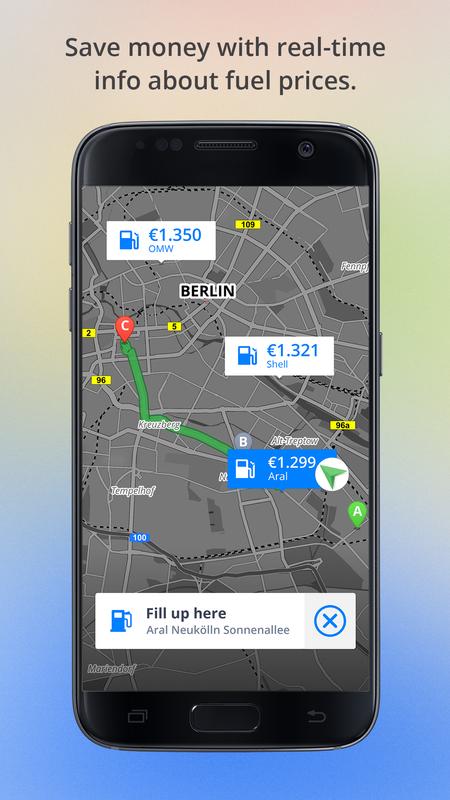This advertisement showcases a mobile application designed to help users save money by providing real-time information about fuel prices. Featured prominently is a smartphone displaying a detailed map of Berlin. 

On the screen, various gas stations are marked with icons representing gasoline pumps, each accompanied by the current fuel prices. Three highlighted stations include OMW, priced at €1.35, Shell at €1.32, and Aral at €1.29. The Aral station is specifically highlighted in blue with the tag "Fill up here," located at Neukölln-Sennenal, indicating it offers the lowest price at €1.29. 

The app's functionality is further illustrated with a blue "X" next to the Aral station, suggesting users can click to receive directions. A pin with the letter "C" in the middle indicates the user's current location. 

The map itself is rendered in shades of gray, featuring light gray, dark gray, and black dotted lines to denote various roads and boundaries. Additional numerical markers in yellow squares, such as 25, 109, and 96, indicate different points of interest or street numbers, adding further detail to the geographic context. This visual representation emphasizes the app's utility in finding the cheapest gasoline prices within Berlin to aid users in making more cost-effective fueling decisions.